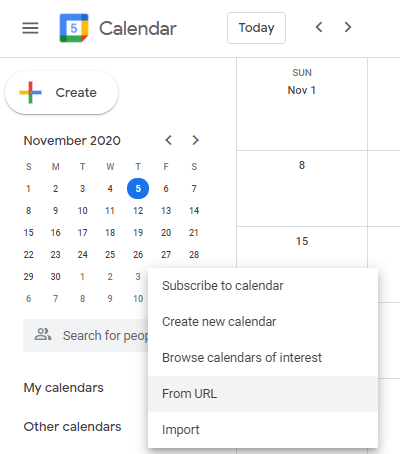The image features a digital calendar interface. At the very top, there is a box displaying three horizontal black lines stacked on top of each other. To the right of these lines is a colorful square divided into blue, green, and yellow sections, with the number "5" prominently displayed inside. Adjacent to this square, the word "Calendar" is written in bold black letters.

Next to the "Calendar" label, there is a white banner containing the word "Today" centered within it. Flanking this banner are two arrows; one pointing left and the other pointing right, signifying navigation options.

Below these elements is the monthly calendar. In the top left corner of this section, there's a colorful plus sign next to the word "Create." Directly below, the text "November 2020" is shown, indicating the month and year. 

The days of the week are displayed in a row beneath this heading, abbreviated as SMTWTFS for Sunday, Monday, Tuesday, Wednesday, Thursday, Friday, and Saturday.

On the actual calendar grid, each Sunday column is marked with the respective date: "Sunday, November 1" is followed by "November 8" and "November 15" in subsequent rows. 

At the bottom of the image, another box appears with various options. These options include "Subscribe to calendar," "Create new calendar," "Browse calendars of interest," "From URL," and "Import."